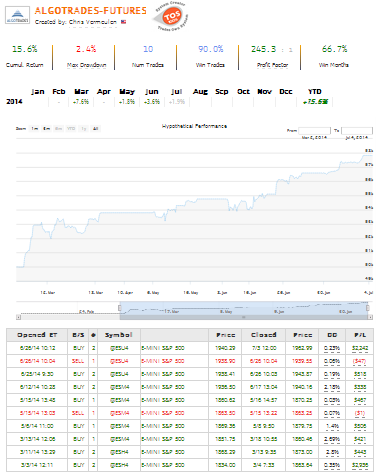This image appears to be a screenshot from a non-English website titled "AlgaTrades/Futures." The background is predominantly white, and a small, unreadable text follows the title, likely indicating the creator or additional details. A logo is displayed immediately after the title, enhancing the branding of the web page.

Below the title, the screenshot features two main graphical elements: a line graph and what appears to be an Excel-like table. The line graph at the top visually represents data changes over time, although the specific data points and textual labels are too small to decipher. Immediately beneath the line graph is the Excel-like table. Although the text within the table is illegible, the layout displays columns labeled with months—January through December—and another column labeled "Year to Date," suggesting a summary of data for the year 2014.

The data entries within the table appear in different colors, predominantly blue and red, presumably to differentiate various metrics or statuses. However, due to the small print, the precise details of these entries remain unreadable. The overall design conveys a structured approach to data presentation, likely aimed at tracking or analyzing trading futures.